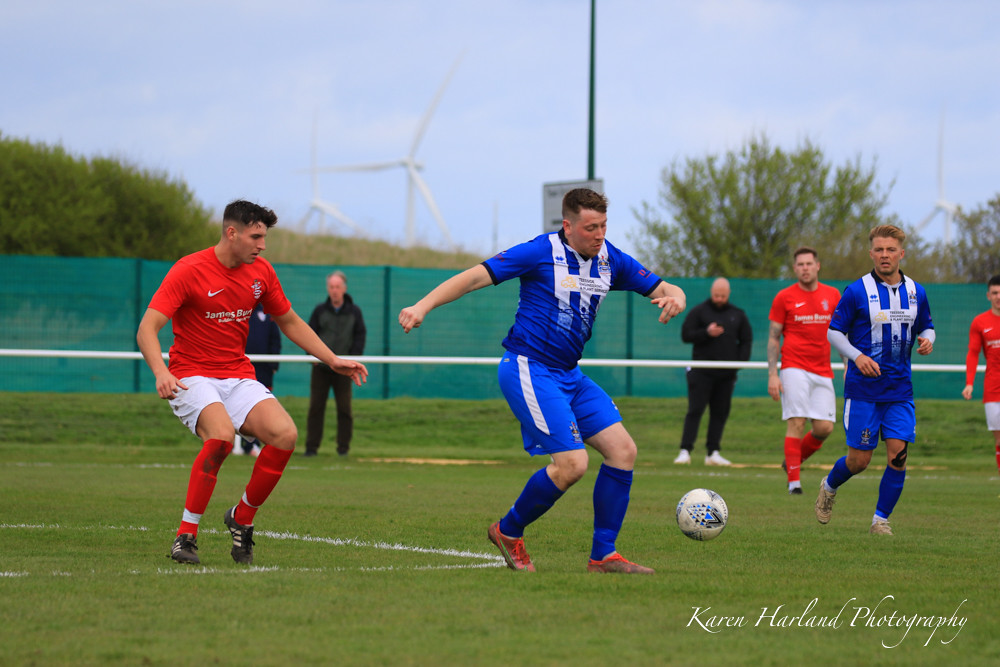In the image, a lively soccer match unfolds on a verdant green field. The scene is dominated by players in red jerseys with white shorts and red socks facing off against opponents in blue jerseys with vertical white stripes, blue shorts, and blue socks. The focal point is a blue-clad player about to kick a colorful soccer ball, while others from both teams are either approaching or defending. A watermark in the bottom right corner reads "Karen Harland Photography" in italic cursive script, identifying the photographer. In the background, spectators, possibly coaches, stand attentively near the field's edge. Beyond them, a green mesh fence borders the field, with a hillside adorned with shrubbery and a trio of wind turbines rising against the clear, blue daytime sky, their white blades contrasting with a few scattered clouds.